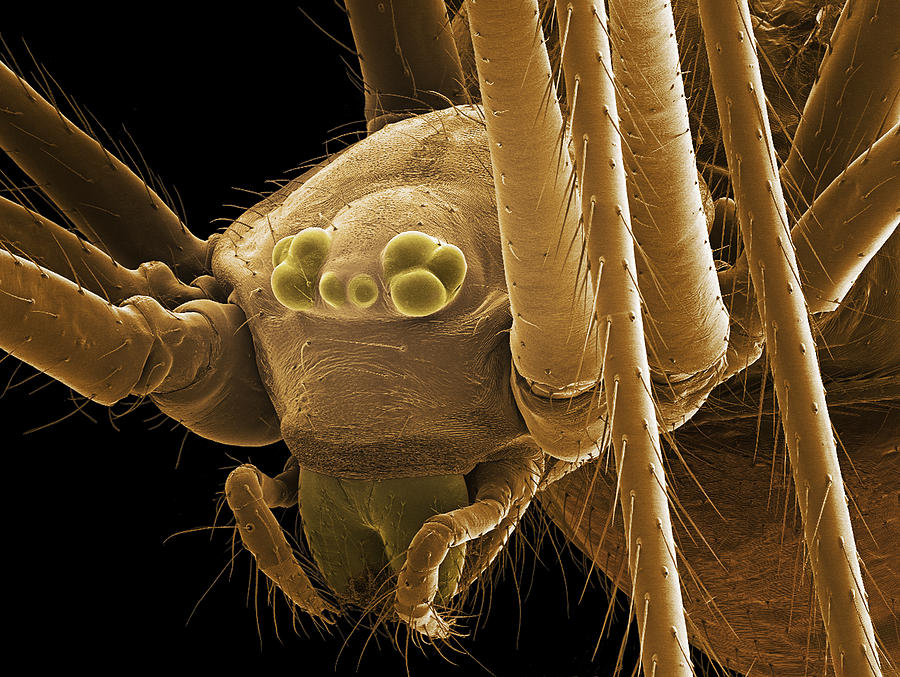This high-definition image is a horizontally rectangular, extremely close-up photograph of a spider, possibly taken with an electron microscope, showcasing the remarkable detail of the arachnid's anatomy. Rendered in a sepia tone, the photo emphasizes the intricate textures and variations in shades, giving the light tan, almost beige spider a dramatic contrast against the dark, black background. The spider's head is prominently centered, capturing its multiple eyes arranged in two sets of three larger eyes with two smaller eyes nestled between them. Below the eyes, you can see its fearsome pinchers, likely used for feeding, flanked by smaller, hairy arms that appear to assist in directing food to its mouth. The spider's legs, bristling with countless hairs, extend towards the left of the image, enhancing the sense of magnified realism. The incredibly sharp resolution highlights the modern, professional quality of the photograph, which seems ideal for scientific research, although it evokes an intimidating and somewhat terrifying impression due to the intense level of detail and the natural aversion many feel towards spiders.